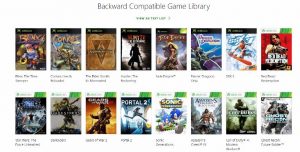This is a very small horizontal rectangular image titled "Backward Compatible Game Library" at the top in tiny text. The image showcases thumbnail previews of various games arranged in two rows, each containing eight thumbnails for a total of sixteen. Due to the small size, the specific titles of the games are unreadable. Each thumbnail tends to have a black horizontal bar at its top, and nine of them feature a small light green rectangular area in the upper right corner, possibly indicating some form of compatibility or special feature. Most game covers depict a person, and there are small, illegible words below each thumbnail, with some text appearing in light green font beneath the title at the top.